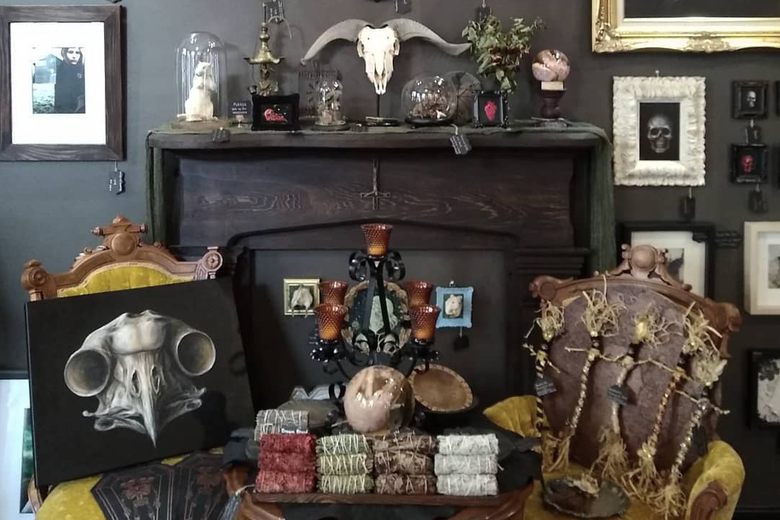The living room depicted in the image presents a captivating collection of curiosities and vintage decor. Dominating the room is a dark gray walled mantel with brown framing, though notably without a fireplace. Instead, the interior of this faux fireplace is adorned with candles in black candlestick holders with orange-brown glass, along with framed pictures, contributing to the eclectic and eerie atmosphere.

Above the mantel sits a striking white skull with long horns, resembling a bison’s head, flanked by various decorative collectibles. Among these, a globe encasing a preserved meerkat stands out, enhancing the room’s oddity charm. The walls around the mantel are adorned with framed art, some featuring skeletal skulls, adding to the room’s macabre theme.

Two ornate, wood-framed vintage chairs with mustard-color velvet upholstery are positioned on either side of the mantel. The chair on the right hosts peculiar twine-made dolls that evoke a sense of witchcraft. The left chair supports a large painting showcasing a bird skull with striking round eyes on a black background, further emphasizing the room’s fascination with skulls and the unusual. 

A coffee table, situated nearby, is scattered with sage sticks, and more art hangs on the walls, including an eerie portrait of a girl. The room's overall atmosphere is a curated display of oddities, where every piece, from taxidermied animals in glass jars to the numerous skull depictions, contributes to a unique and intriguing aesthetic.